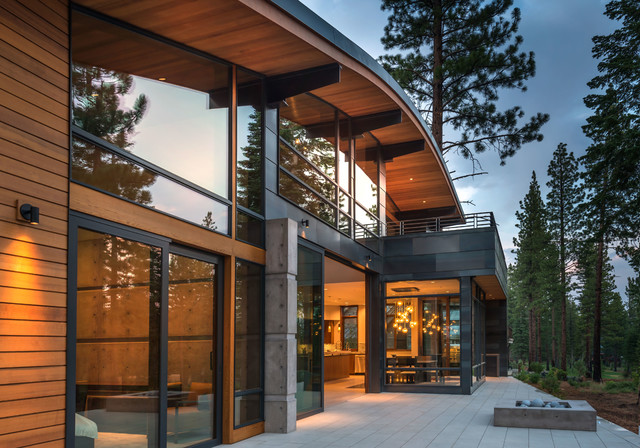This detailed photograph captures a large, luxurious house with modern architectural elements, nestled against an evergreen forest with a sky that hints at dawn or dusk in a grayish-blue hue. The central focus is the house’s extensive glass facade, which provides a glimpse into a tastefully decorated interior featuring tables, kitchen area, and possibly a bedroom. The exterior showcases a combination of horizontal golden-wooden siding, black metal accents, and expansive glass windows. The curvature and structure of the house are complemented by an upper deck above the kitchen area and a black metal balcony. A gray-tiled patio extends outwards, where a square stone fire pit with rocks can be seen in the lower right corner. Several tall pine trees rise in the background, adding to the serene, upscale mountain retreat feel of the residence. Bright, dangling lights inside the house and the reflection of trees and the sky in the windows add to the picturesque quality of the photo.